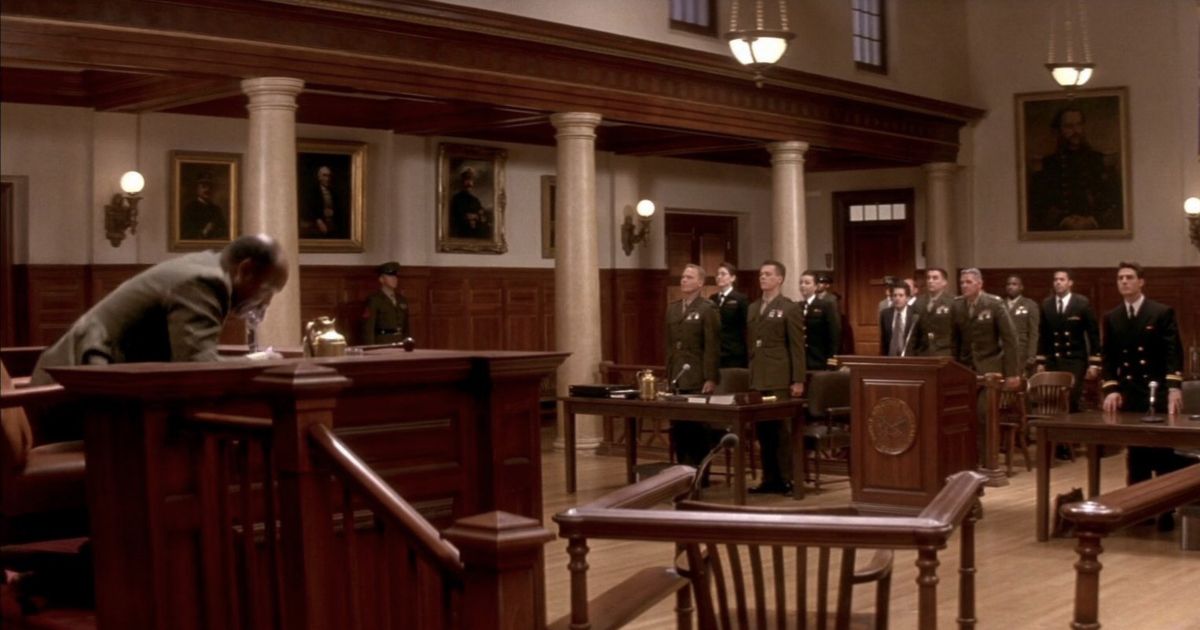The photograph captures an ornate and old-fashioned courtroom, likely military, with dark brown wood paneling, white marble columns, and hanging chandeliers. The gallery, adorned with historic portraits and a large picture on the back wall, houses a group of men, all with similar haircuts and predominantly in military uniforms, either dark army green or black. In the forefront, a partially bald man in a gray suit leans over a high-backed chair at a podium, with a golden mug or vase on the desk before him. The scene is meticulously detailed with elements such as light fixtures, wooden banisters, and a polished wooden floor, giving it a timeless, almost historical ambiance.